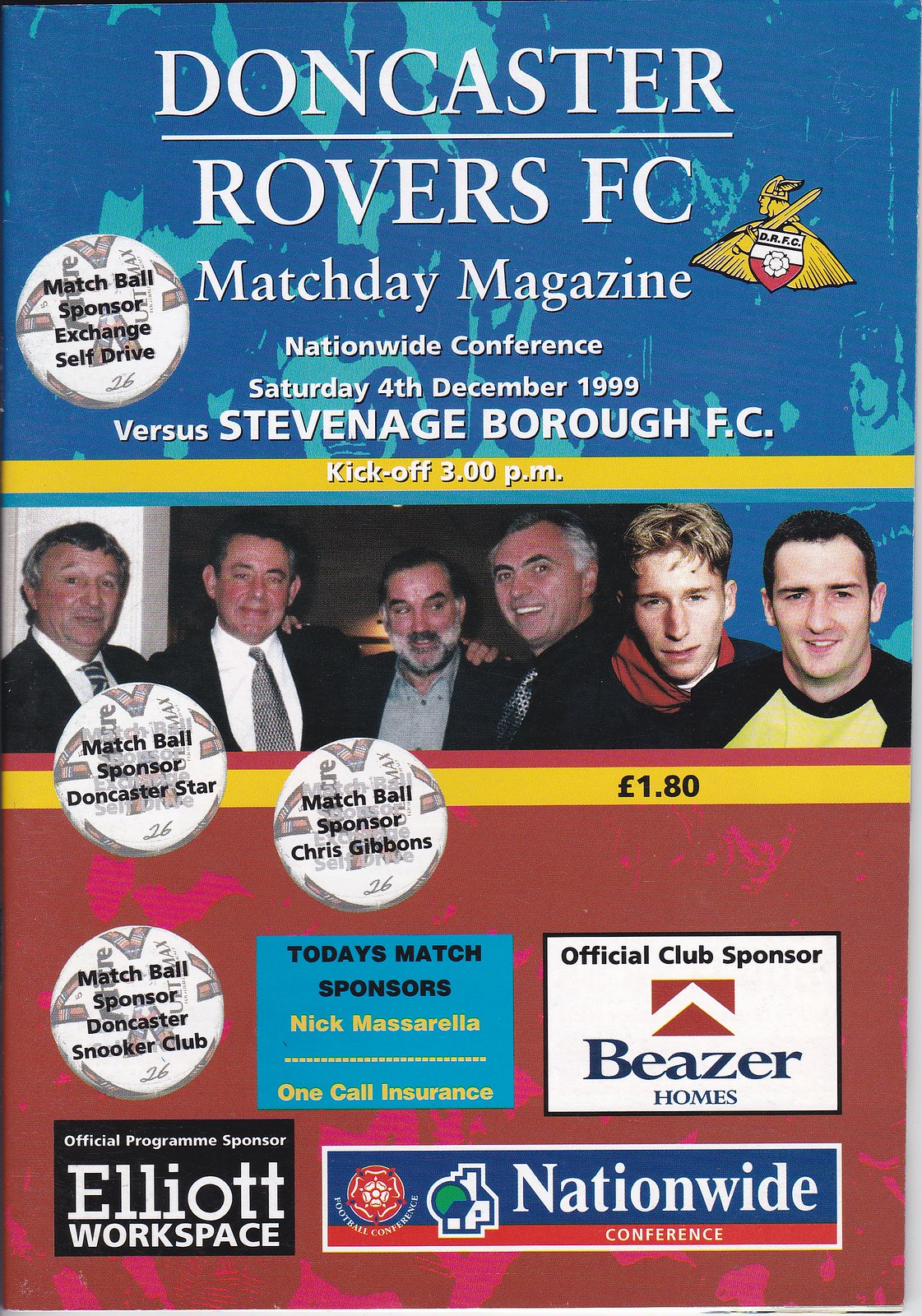The image is the front cover of a Doncaster Rovers FC Match Day Magazine for a soccer match. The top third of the cover features a blue and white background with the text "Doncaster Rovers FC, Match Day Magazine, Nationwide Conference, Saturday 4th December 1999, versus Stevenage Borough FC" prominently displayed. Below this, there is a yellow stripe with white lettering indicating "Kick off 3pm." In the center of the cover, there is a banner showing a photograph of six men standing side by side. Directly beneath this, there is another yellow stripe with black text displaying the price, "£1.80." The lower section of the cover has a red background and showcases various sponsor logos, including Nationwide Conference, One Call Insurance, and Beezer Homes. Additional sponsorship details, such as "Match Ball Sponsor: Chris Gibbons" and "Official Club Sponsor: Beezer Homes," are also included. The cover is vibrant, featuring a mix of colors like blue, red, yellow, black, and white, with numerous smaller advertisements and labels displaying different sponsors and companies.